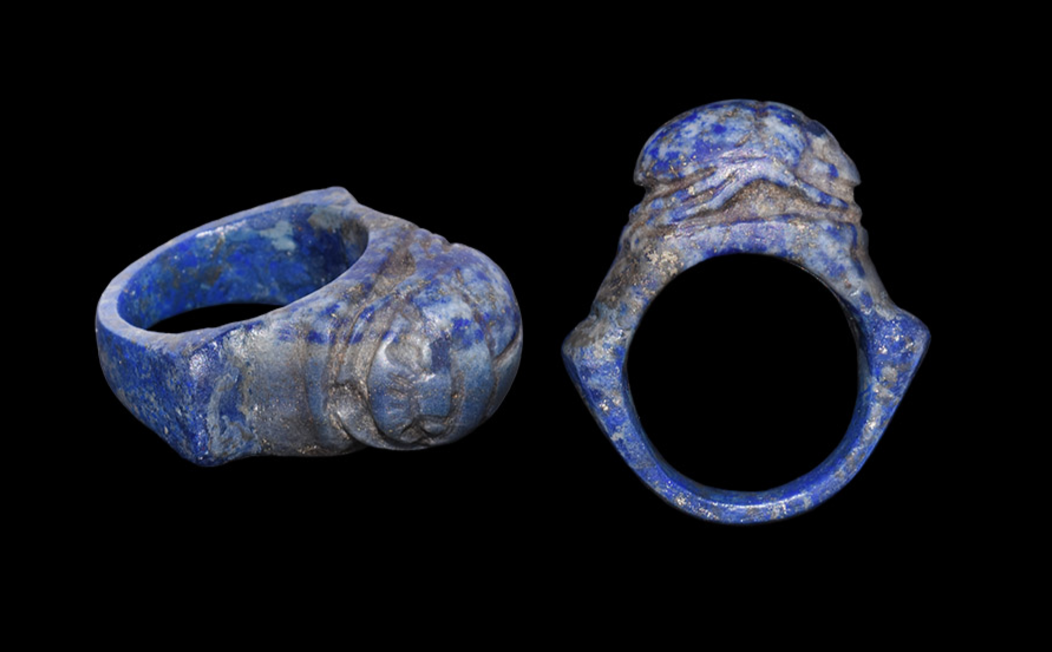The photograph showcases two ancient-looking rings positioned against a stark black background, possibly a sheet of black paper approximately four by six inches in size. The rings, predominantly blue with shades of gray and potential signs of rust, appear to be crafted from stone. Each ring is adorned with a bulb-like feature, and one ring, viewed from a specific angle, reveals a hole at the center with a top resembling muslin fabric and ridged edges. These rings, with their intricate designs and weathered appearance, suggest they hail from an ancient civilization, though their exact origin remains unknown. The stark simplicity of the setting emphasizes the uniqueness and antiquity of these beautiful artifacts.